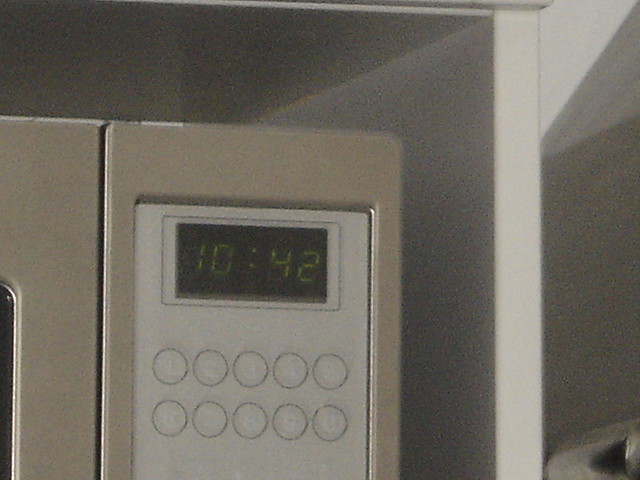This image portrays a close-up, slightly blurry photograph of the top right-hand corner of an older, beige microwave. The device is digitally equipped, featuring a black horizontal display with green lit digits that read "1042," indicating either the current time or the duration of cooking. Below the display are two rows of ten numbered buttons, though the numbers appear worn. The microwave is slotted into a white cabinet or shelf, likely within a home or dorm kitchen. The lighting in the room is dim, casting subtle shadows across the microwave, adding to its aged and somewhat dingy appearance. No people are present in the image.